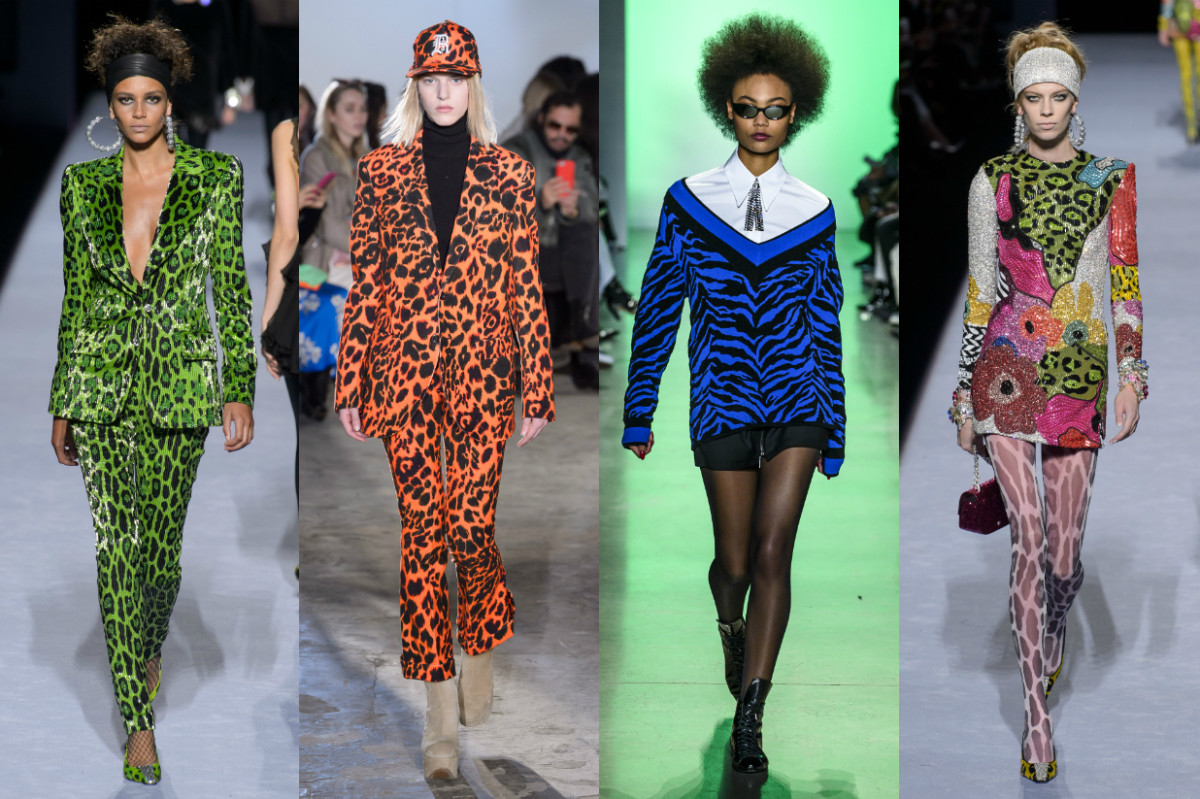This image features four vertically aligned photos of runway models showcasing eclectic fashion ensembles. The first model is an African American woman with dark, curly hair styled away from her face with a thick black head wrap. She sports large silver hoop earrings and a striking green cheetah print pantsuit, worn without a shirt but complemented by a matching sport coat and heels. The second model is a blonde, white woman adorned in an orange animal print ensemble, complete with a suit coat, cropped trousers, and a matching baseball cap. She pairs this striking look with a black turtleneck and tan boots, capturing the attention of an ambient backdrop filled with spectators taking photos. The third model, another black woman with an afro hairstyle and glasses, showcases a white Peter Pan collared shirt accented with a cravat, layered under a blue and black animal print sweater draped off one shoulder. She completes her look with black shorts, black pantyhose, and boots, strolling against a green-tinted runway background. The fourth model, a blonde white woman, accessorizes her messy bun with a thick white headband and large hoop earrings. She wears a dazzling dress featuring an eclectic mix of animal prints, florals, and sparkles, along with giraffe print pantyhose and a maroon handbag, pulling her vibrant look together.